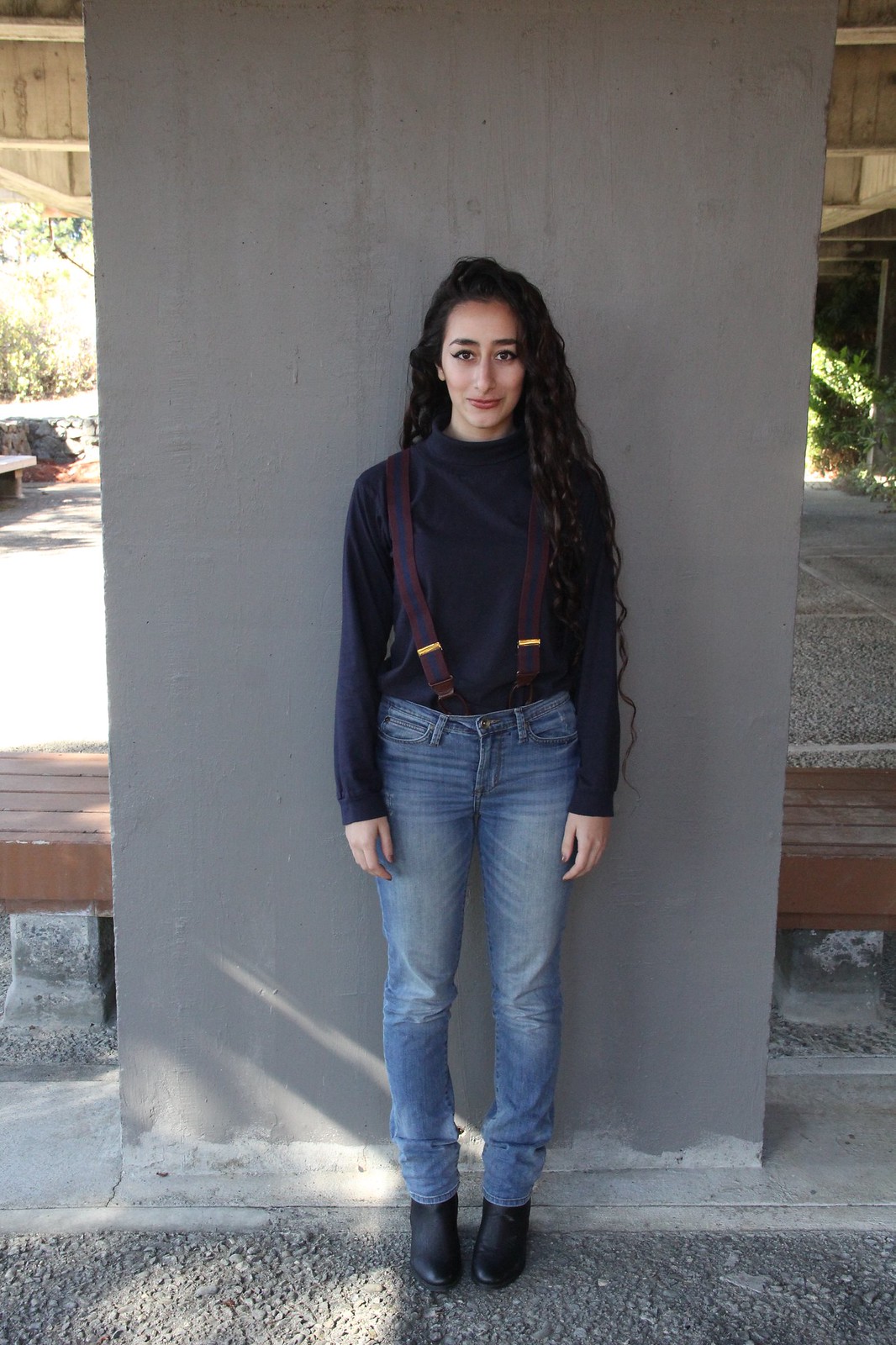In this photograph, a woman stands against a wide, gray concrete pillar in what appears to be an underground parking garage. The pillar, about six feet wide, has wooden benches extending from either side. To the right of the pillar, the parking area is visible with painted lines marking parking spaces. On the left, another bench and a short rock wall with greenery above are in view. The ground is gray and rocky, giving the area a gritty texture. The woman, positioned with her feet on this rough surface, has long, curly hair parted to the left side and falls almost to her back. She gazes directly at the camera with a slight smile and wears black eyeliner. Her outfit includes a black long-sleeve sweater, maroon suspenders with a hint of gold at the ends, blue jeans, and black boots. Both of her hands rest at her sides, capturing a casual yet poised stance.